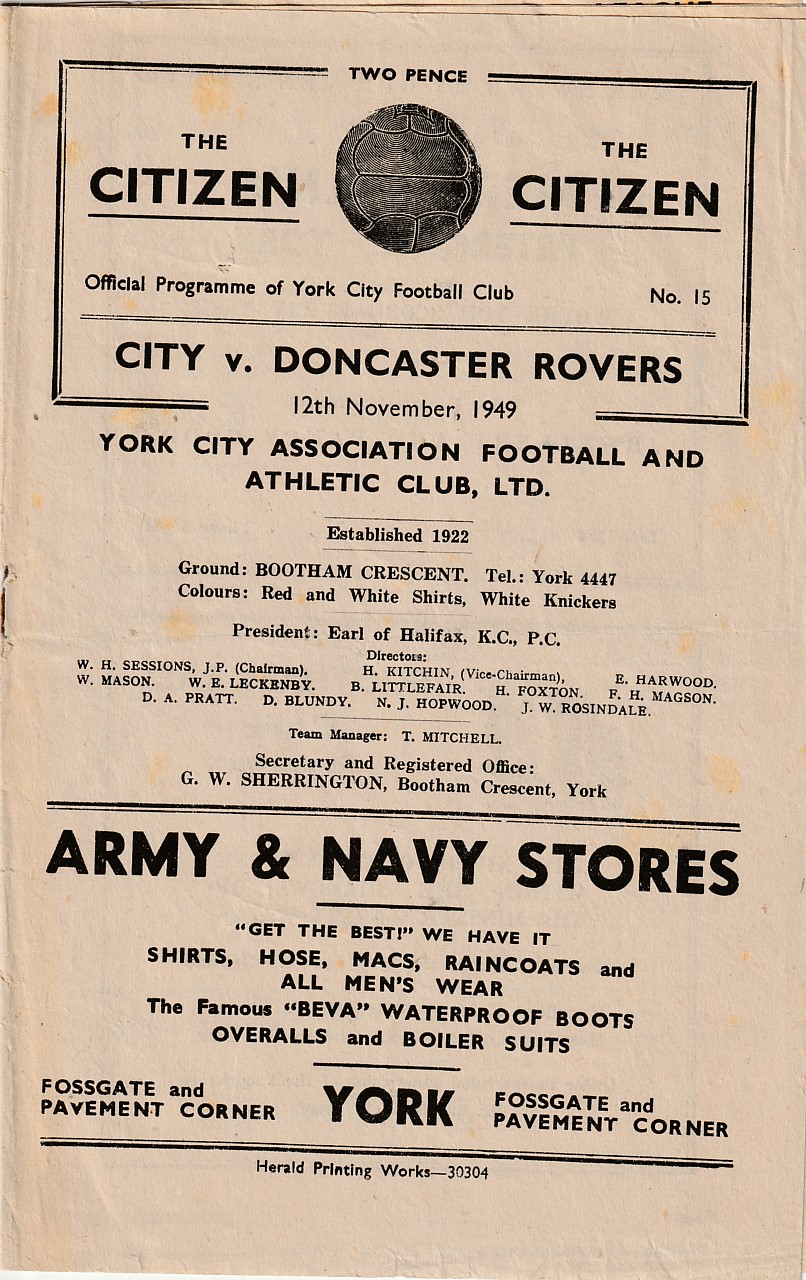This image captures a vintage poster or program cover dated November 12, 1949. At the top, it reads "Two Pence" and prominently features "The Citizen" on both the left and right sides of a central globe-like emblem. Below, it states "Official Program of York City Football Club No. 15" with an underlining line. The event detailed is "City V Doncaster Rovers" held on the mentioned date. Further down, it includes "York City Association of Football and Athletic Club, LTD, established 1922, Ground Bootham Crescent, Telephone: York 4447" and mentions the team colors: "red and white shirts, white knickers." The president is listed as "Earl of Halifax, KC, PC," followed by an illegible list of directors' names. 

An advertisement for "Army and Navy Stores" dominates the bottom, boasting slogans such as "Get the Best – We Have It," along with products like "shirts, hose, macs, raincoats, and all menswear," including the "famous Beaver waterproof boots, overalls, and boiler suits," located at "Fosgate and Pavement Corner, York." Finally, the bottom right corner states "Herald Printing Works, 30304."